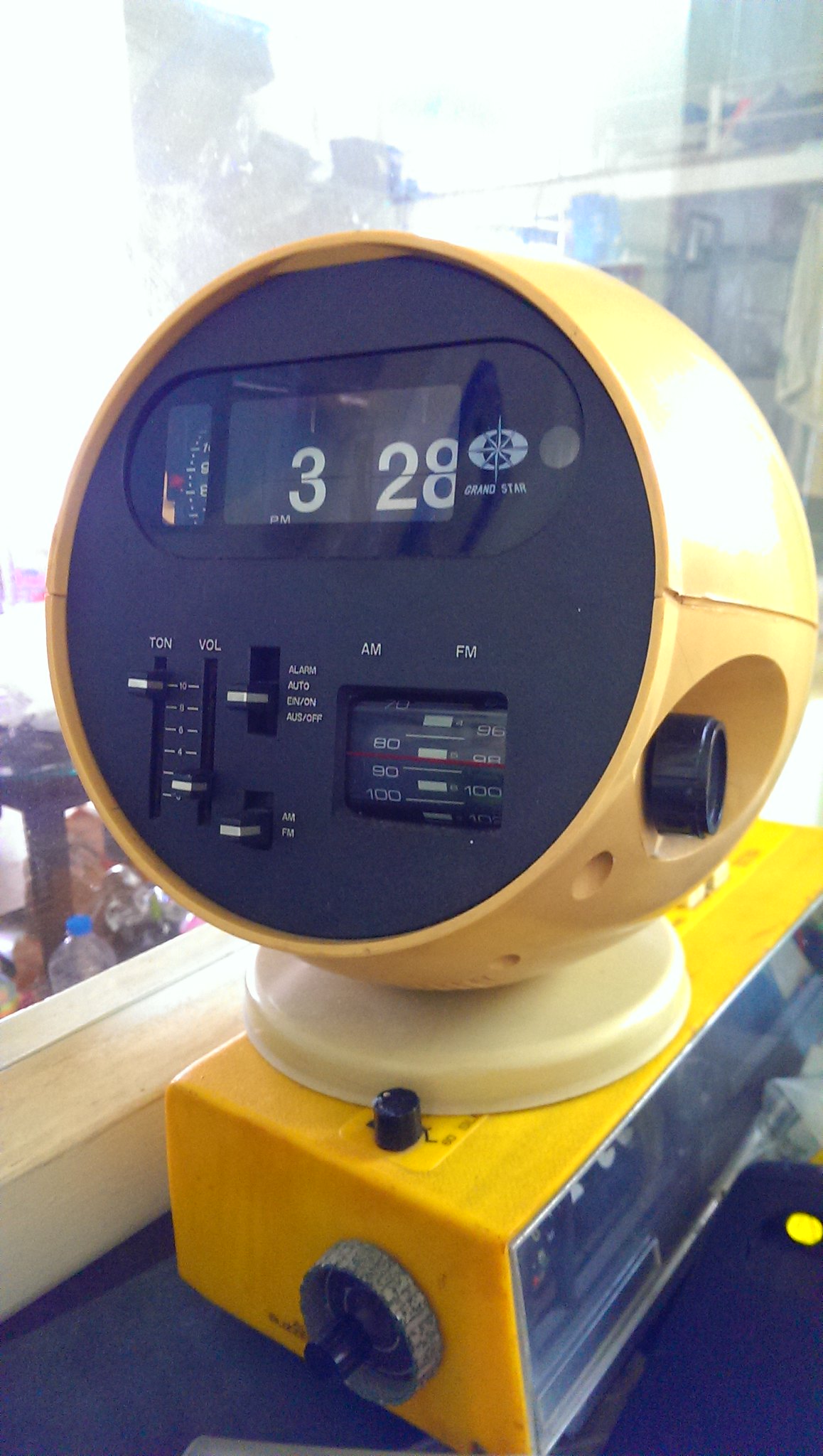This photograph captures a unique arrangement of two clocks stacked one on top of the other. The top clock features a round, plastic casing with a black face and white numerals, displaying the time as 3:28. This clock also functions as a radio, complete with a black tuning knob on the side for adjusting stations between AM and FM, and several levers for volume and other settings. It is balanced on a flat, cream-colored base. Below it sits a bright yellow, rectangular clock, also plastic, with a black knob and a black face, although the time on this clock is not legible. This bottom clock appears old, worn, and slightly dirty, contrasting with the relatively modern look of the clock above.